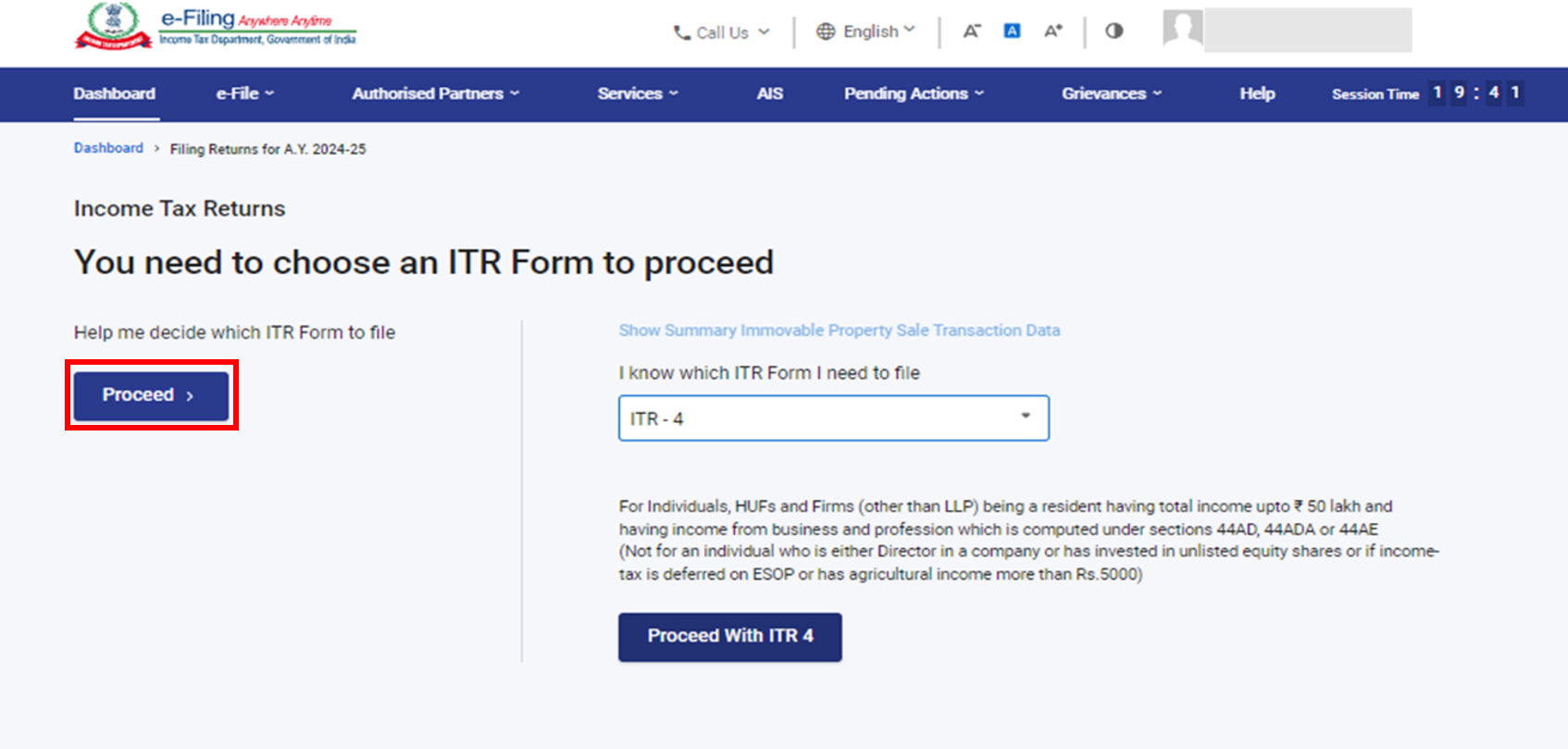**Detailed Caption:**

This image is a screenshot of the Income Tax Department’s official website for e-filing tax returns in India. In the upper left-hand corner, there's a governmental seal adorned in green, red, and blue hues. Adjacent to the seal, the text "e-Filing Anywhere Anytime" stands out in blue and red, followed by "Income Tax Department, Government of India." To the right of this header, there is a section providing contact information, language options, font preferences, and various login choices.

Directly beneath this header runs a blue navigation bar with white text displaying several options: Dashboard, e-File, Authorized Partners, Services, AIS, Pending Actions, Grievances, Help, and a session timer currently showing "Session Time: 1941." Below the navigation bar, there is a light gray box designed to guide users through the Income Tax Return (ITR) filing process. 

The gray box includes multiple smaller fields and instructive text, stating: "Income Tax Returns: You need to choose an ITR form to proceed." There is a blue button labeled "Proceed" highlighted in red to prompt user action. To the right, a drop-down menu is present with the text, "I know which ITR form I need to file," currently set to ITR 4. Alongside this, there's another blue rectangular button with white text labeled "Proceed with ITR 4," facilitating the user's filing process.